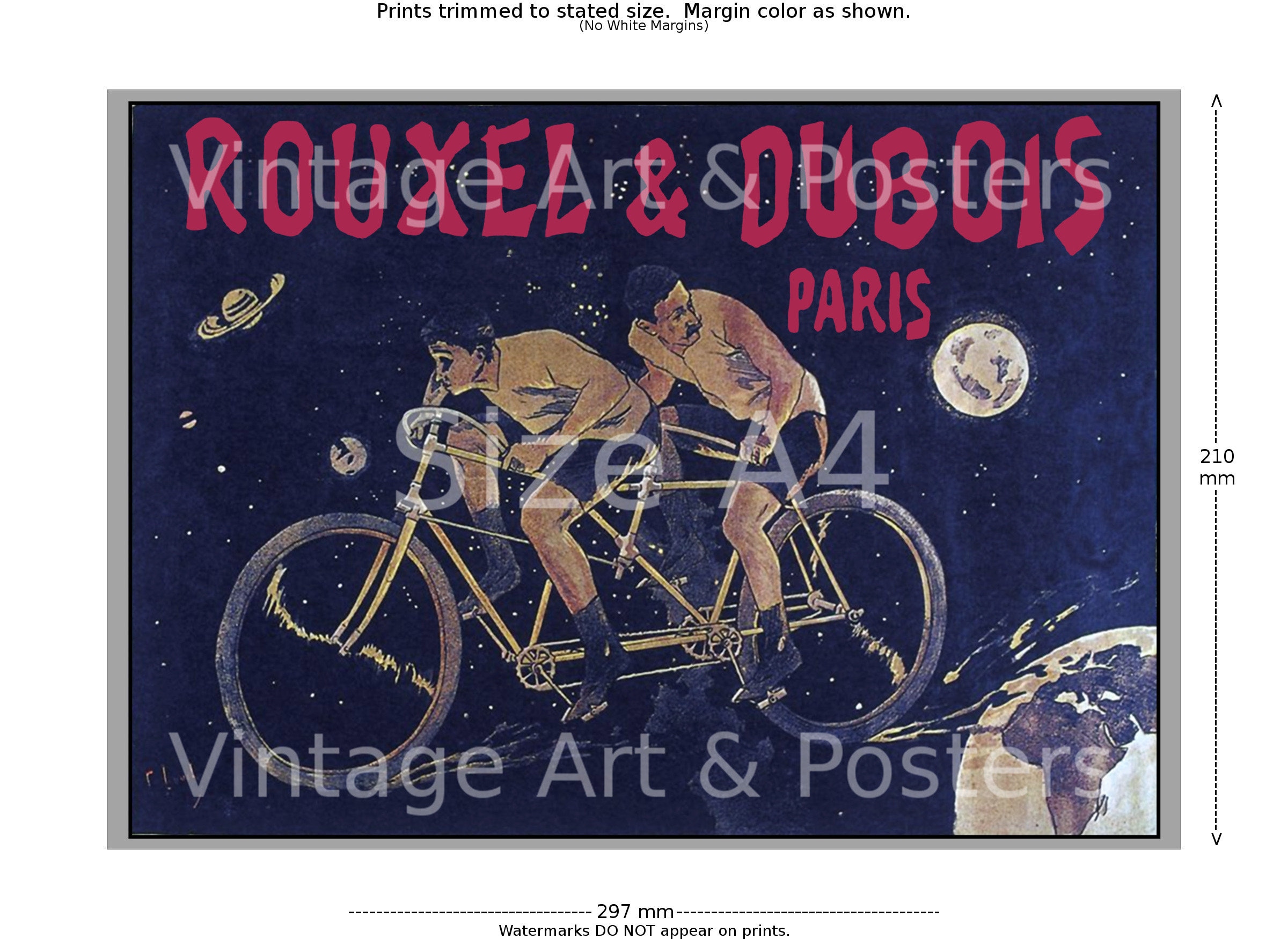This horizontally oriented, graphic poster showcases a whimsical painting of a tandem bicycle with two men in old-fashioned attire, both clad in yellow shirts, black shorts, socks, and shoes. They are depicted riding through an outer space scene, with the Earth positioned in the lower right corner and Saturn, the Moon, and other stars spread across the celestial backdrop. The upper and lower borders of the poster prominently feature the phrase "Vintage Art and Posters," which is also repeated in French, with "Paris" written underneath in red text. Additionally, the poster is outlined with dimensions: 297 millimeters wide and 210 millimeters high. Annotations outside the poster clarify that prints are trimmed to the stated size, with the margin color as shown and no white margins. There are also watermarks on the image that do not appear on actual prints.